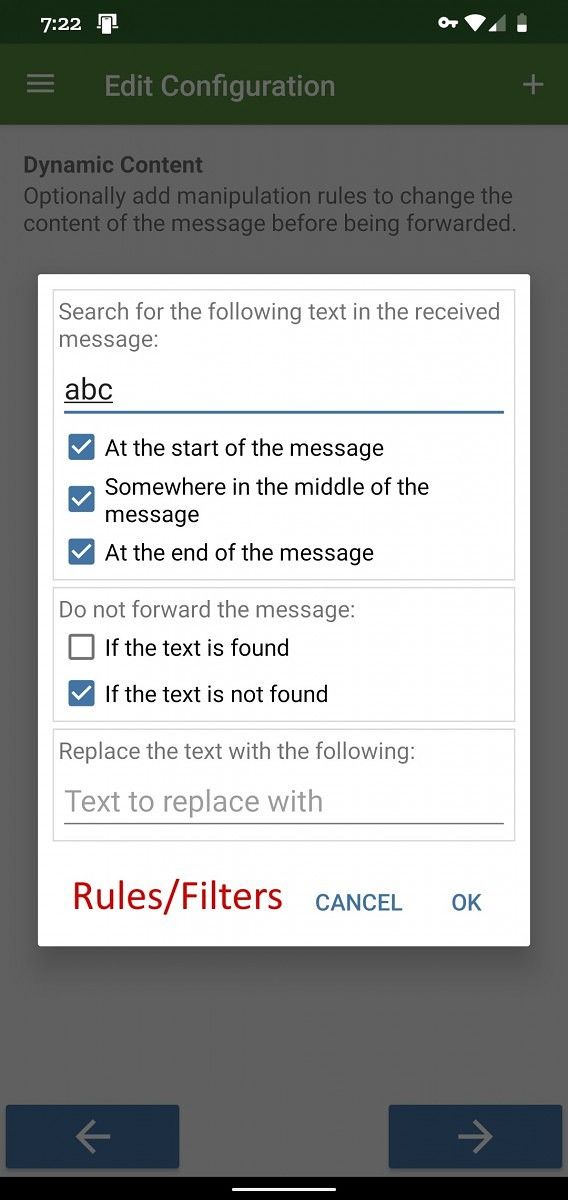Here is a cleaned-up and detailed caption for the described image:

---

The image depicts an iPhone screen with a semi-transparent gray overlay, partially obscuring the underlying content. At the top of the screen, "722" is displayed, indicating the time, with various status icons aligned on the left and right, including a battery icon that is approximately half-filled.

Centered on the screen is a pop-up configuration window with multiple sections:

1. **Header Section:**
   - Text: "Edit Configuration"
   - Sub-header: "Dynamic Content"

2. **Middle Section:**
   - A descriptive prompt: "Search for the following text in the received message."
   - An underlined search term: "ABC"

3. **Search Location Options:**
   - "At the start of the message" 
   - "Somewhere in the middle of the message" 
   - "At the end of the message"
   Each of these options has a blue box with a checkmark next to it, indicating selection.

4. **Action Options:**
   - "Do not forward the message if the text is found"
   - "If the text is not found" (accompanied by a checked blue box, indicating it is the active condition)
   
5. **Text Replacement Section:**
   - Instructions: "Replace the text with the following", followed by a blank input field labeled "Text to replace with".

6. **Footer Section:**
   - In red text: "Rules/Filters"
   - Cancel button labeled "CANCEL" in blue, and an "OK" button in blue next to it.

The gray overlay suggests that the configuration window is superimposed on an underlying webpage, temporarily disabling interactions with the content beneath.

---